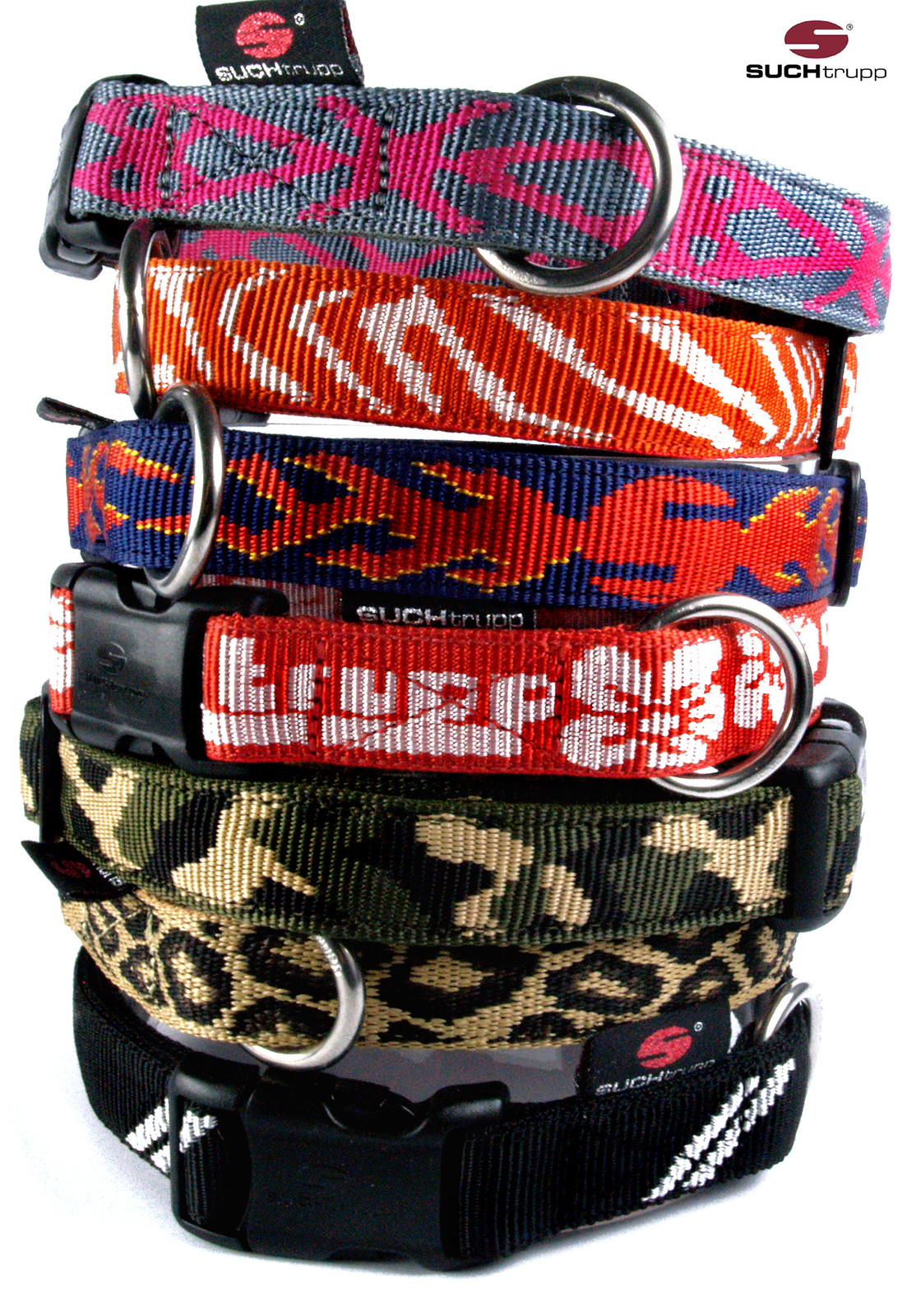The image showcases a stack of dog collars against a plain white background. At the top, a gray collar with a pink geometric design is visible, followed by an orange collar adorned with white patterns. Below it is a navy blue collar featuring red and yellow flame motifs intertwined with S-shaped patterns. The next collar is red with distinctive white text and floral designs. Beneath this, a traditional green camouflage collar combines olive green, black, and tan hues. Further down is a tan collar with a black cheetah print. At the bottom, there is a black collar with subtle white accents. Each collar is equipped with metal rings for tags and black plastic clasps. The image also includes a logo in the upper right-hand corner: an emblem with an "S" above the words "such TRUPP."